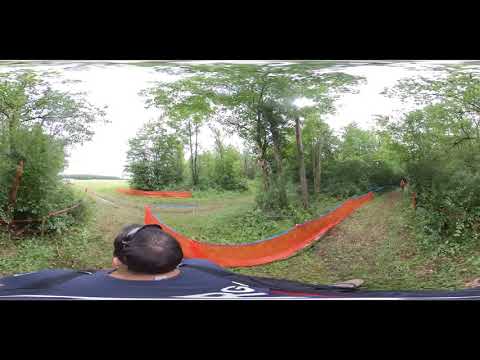This image captures a 360-degree view of an outdoor setting, featuring a somewhat distorted panorama. At the lower left portion of the image, you can see the back of a Caucasian person’s head with dark brown hair, adorned with sunglasses resting on top. The individual is wearing a dark blue t-shirt with partial letters “R” and “G” visible. Standing directly in front of the camera, they appear to be walking along a trail.

The scene depicts two rows of short, orange netted fences, suggesting an area marked off, potentially for a dirt bike or motorbike path. The dirt road that runs through this space is surrounded by dense greenery, consisting of bushes and scraggly, non-landscaped trees, with larger trees appearing both at the center and to the left of the image.

Additionally, the background reveals a blend of cyan sky and white clouds, indicating a sunny day with some cloud cover. The natural, brushy environment enhances the sense of rugged outdoor adventure, hinting that this could be a place for racing or trail activities.